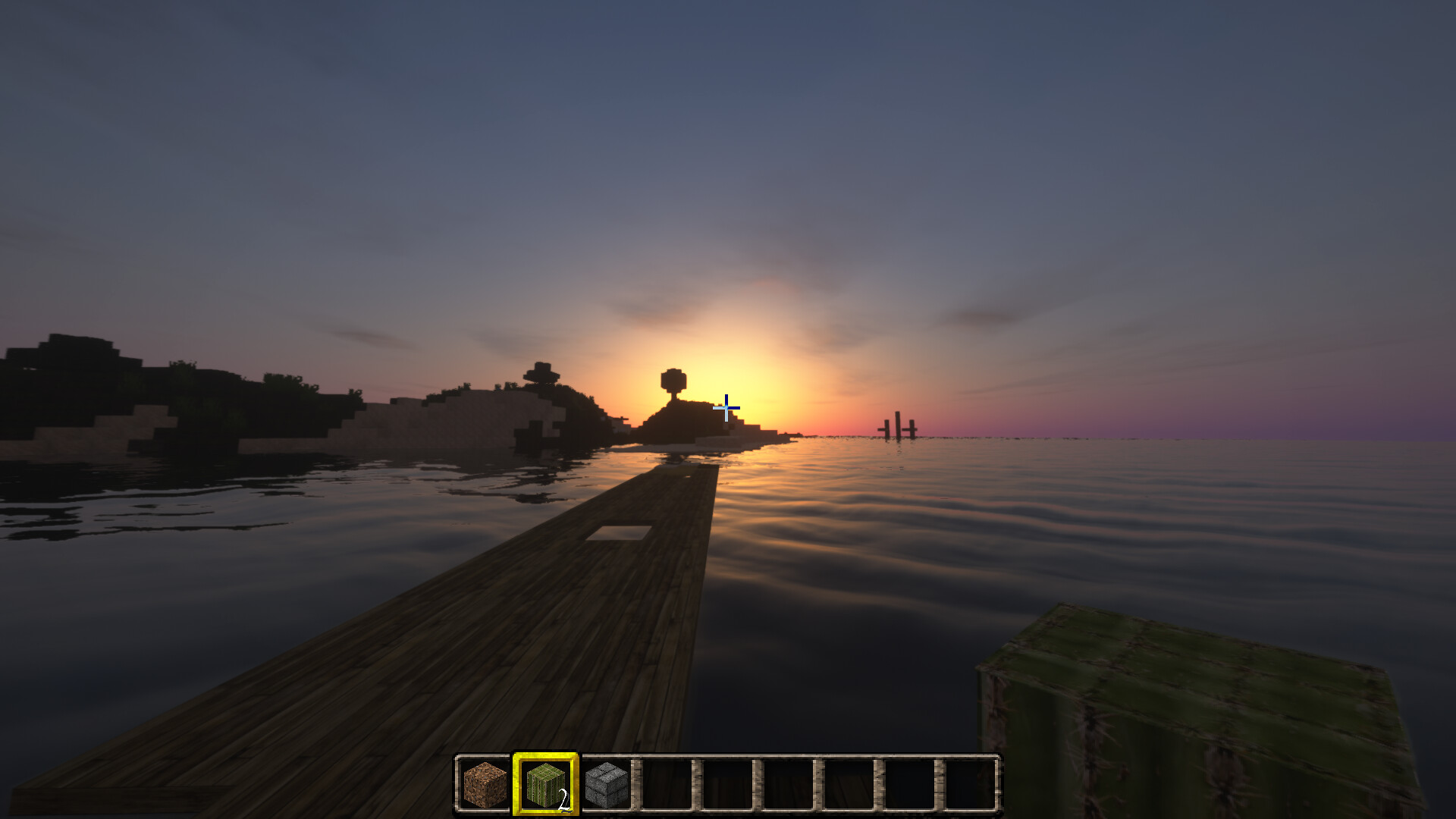The image, a low-resolution screenshot from a PC game, depicts a serene sunset scene viewed from the base of a wooden pier that stretches into a rippling body of water. The central focus is a bright orange-yellow sun setting behind hills, casting an explosion of gold and peach hues that blend into deeper purples and blues across the sky. Faint cloud shadows are also visible, adding to the scenic beauty. To the left, the silhouette of an island structure with darkened tree lines and the outline of buildings is noticeable, while mountains and hills create a backdrop on the horizon.

At the bottom of the screen, there's an item counter consisting of nine outlined squares, the first three containing three-dimensional cubes: a brown one, a green one, and a gray one, followed by six black squares. The green cube’s square is highlighted in yellow. A small green treasure chest is located in the bottom right corner, partially in the water. A tiny X or plus sign sits precisely in the center of the image, likely as a game cursor or focal point. The overall composition beautifully showcases the interplay of natural elements and game design.